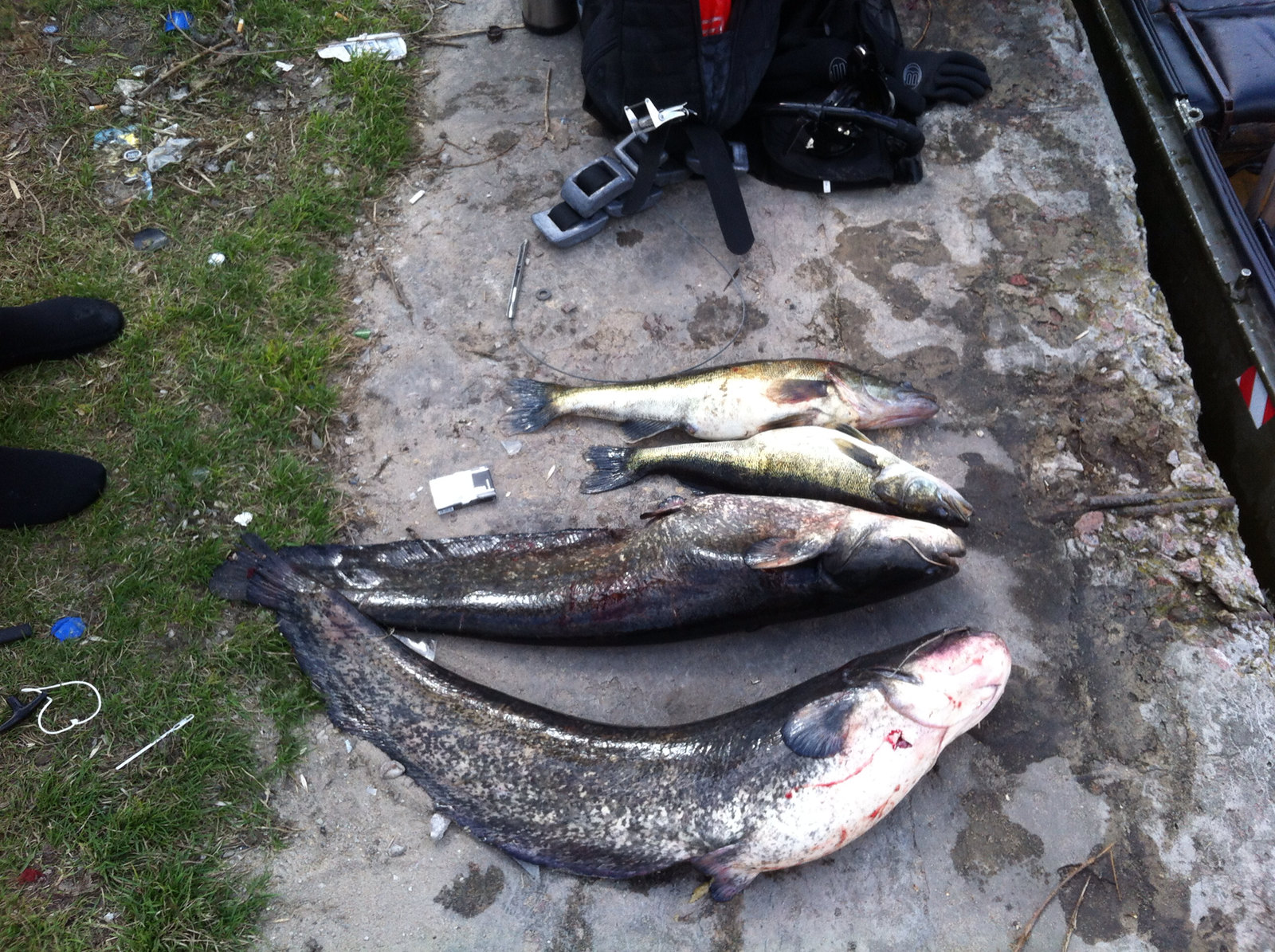This color landscape photograph captures four recently caught fish arranged on a strip of concrete near the edge of a dock. The right two-thirds of the image showcases the concrete surface, while the left third reveals a grassy area and a pair of feet clad in black socks, likely belonging to the person who caught the fish. The four fish, silver with gray bodies, are positioned with two larger fish (approximately two feet long) in the foreground and two smaller fish (around one foot long) in the background. The largest fish at the bottom of the frame is slightly arced, and one of the fish appears somewhat bloody. Surrounding the fish, in the upper center of the photograph, are pieces of equipment, possibly snorkeling or diving gear, with visible black straps and silver-gray buckles. The presence of a black backpack and a pack of cigarettes adds to the scene. Notably, on the right-hand side of the photo, there's a visible gap between the concrete and a gray metal boat, distinguished by a red and white diagonal diver's flag decal. This detailed composition suggests a recent fishing activity right beside the dock.